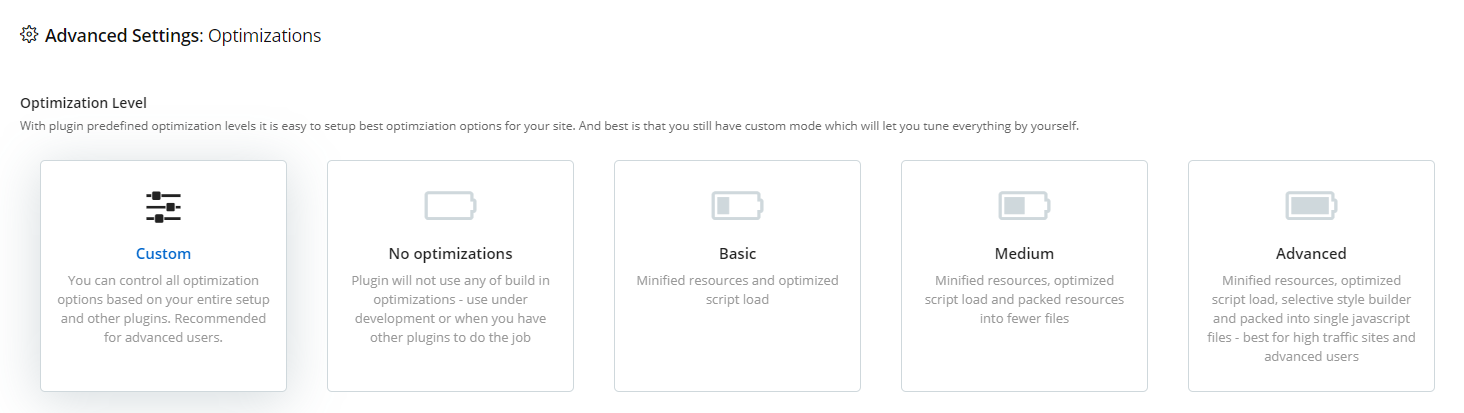A descriptive caption for the image could be:

---

This is a screenshot of a device settings interface, specifically focused on optimization levels. In the top left corner, there is a settings gear icon. To its right, the header reads "Advanced Settings Optimizations." Below this header, a section labeled "Optimization Level" explains the user can easily set up optimization options using predefined levels or a custom mode for personalized adjustments.

The interface features five tiles representing different optimization modes:

1. **Custom**: This tile is selected and features an icon of three sliders at different positions. The label reads "Custom" in blue text. It states that users can control optimization options based on their entire setup and other plugins, recommended for advanced users.

2. **No Optimizations**: Featuring an empty battery icon, this tile indicates that the plugin will not apply any built-in optimizations. It is suggested for use during development or when other plugins handle optimizations.

3. **Basic**: Marked by a battery icon filled at about a quarter, this level offers minified resources and optimized script load.

4. **Medium**: With a half-filled battery icon, this setting includes minified resources, optimized script load, and consolidates resources into fewer files.

5. **Advanced**: Represented by a fully charged battery icon, this comprehensive level provides minified resources, optimized script load, selective style builder, and packs resources into single JavaScript files. It is ideal for high-traffic sites and advanced users.

This detailed interface allows users to tailor their optimization settings according to their specific needs and technical capability.